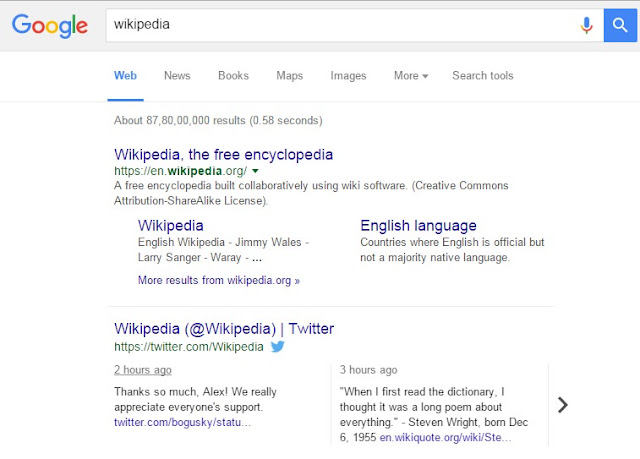**Detailed Descriptive Caption for a Google Search Page Image:**

The image showcases a Google search results page categorized under websites. Positioned at the top left corner is the iconic Google logo, featuring the sequence of colors: a blue 'G', a red 'O', a yellow 'O', a blue 'G', a green 'L', and a red 'E'. The search query entered in the search bar is "Wikipedia". To the right of the search bar is a microphone symbol, indicating the option for voice-to-text input. Additionally, there is a small blue box containing a white magnifying glass icon that represents the search button.

Below the search bar is a horizontal menu with the category "Web" highlighted. Other options in the menu include "News", "Books", "Maps", "Images", "More" with a dropdown arrow, and "Search tools". The largest result on the page is for "Wikipedia, the free encyclopedia", along with a brief description: "a free encyclopedia built collaboratively using wiki software under a Creative Commons Attribution-ShareAlike License."

Further details from the search specify "Wikipedia" followed by subheadings such as "English Wikipedia", and prominent co-founders "Jimmy Wales" and "Larry Sanger". Below this are more results from "wikipedia.org", including content about "English language" and "countries where English is official but not a majority native language."

At the bottom of the page are recent tweets from Wikipedia's official Twitter account. One tweet from 2 hours ago expresses gratitude: "Thanks so much Alex, we really appreciate everyone's support." Another tweet from 3 hours ago features a humorous quote by comedian Stephen Wright: "When I first read the dictionary, I thought it was a long poem about everything."

This organized layout and color-coded design create a user-friendly interface typical of Google search results pages.